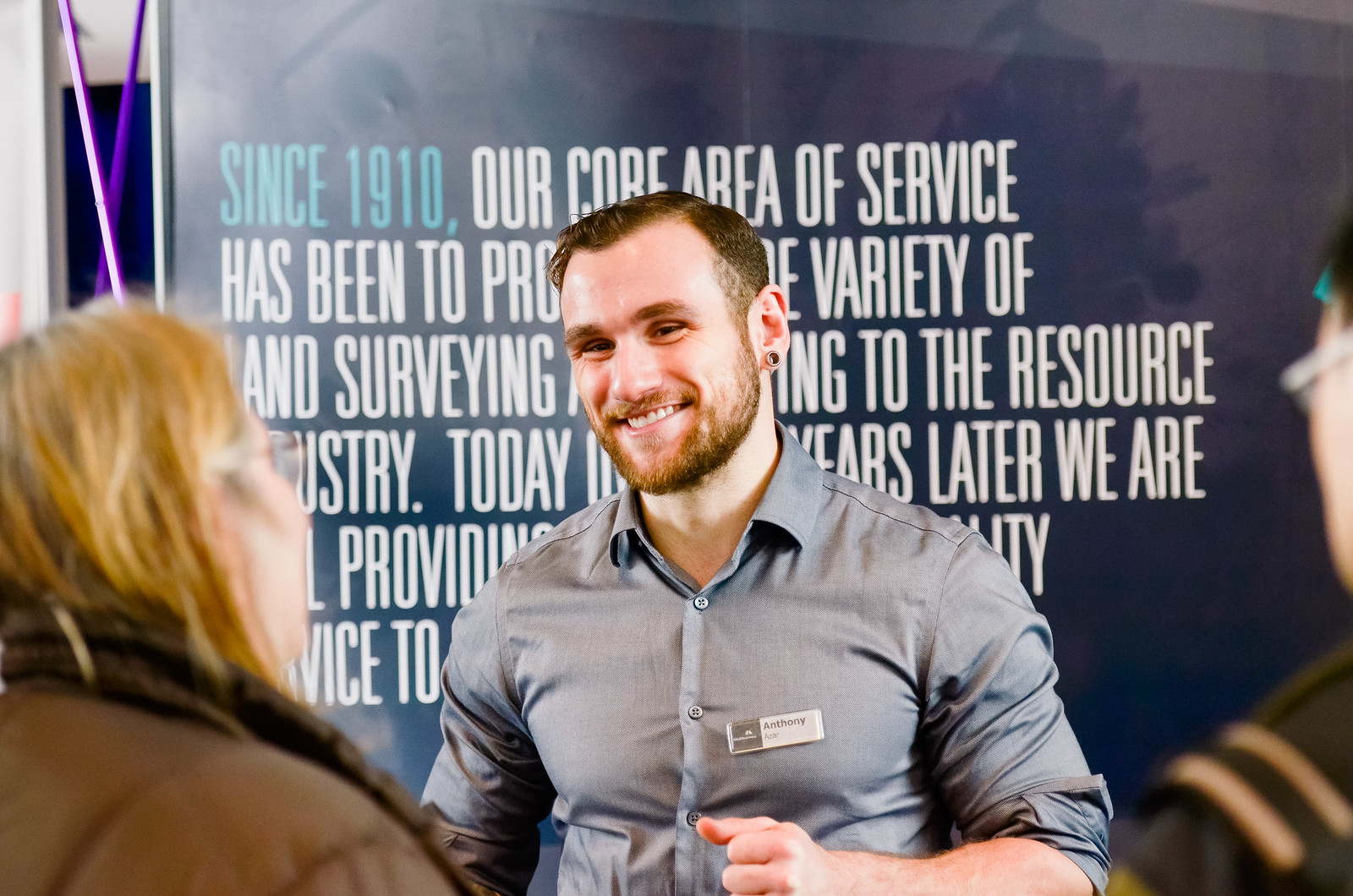The image shows a well-built, Caucasian man in his 30s named Anthony Azar, standing at an event. He is dressed in a tight-fitting, long-sleeve, gray button-up shirt with his sleeves rolled up to the elbow, showcasing his muscles. Anthony has short, reddish-brown hair that is slightly balding and slicked back, and he sports a well-groomed beard and mustache. His nametag is visible on the left side of his chest, where it is gray on the left and white on the right. Anthony is smiling as he engages in conversation with two people. To his left is a woman with long blonde hair, glasses, and a brown puff jacket, who is partially out of frame. To his right, a man with short black hair, glasses, and a brown coat featuring stripes on the shoulder is also visible, though only slightly. The backdrop of the scene is a large blue banner with white writing, featuring the prominent phrase, "Since 1910." The rest of the text is partially obscured by Anthony, making it hard to discern in full. Anthony's positioning and the banner behind him indicate that this is likely a formal event or gathering.